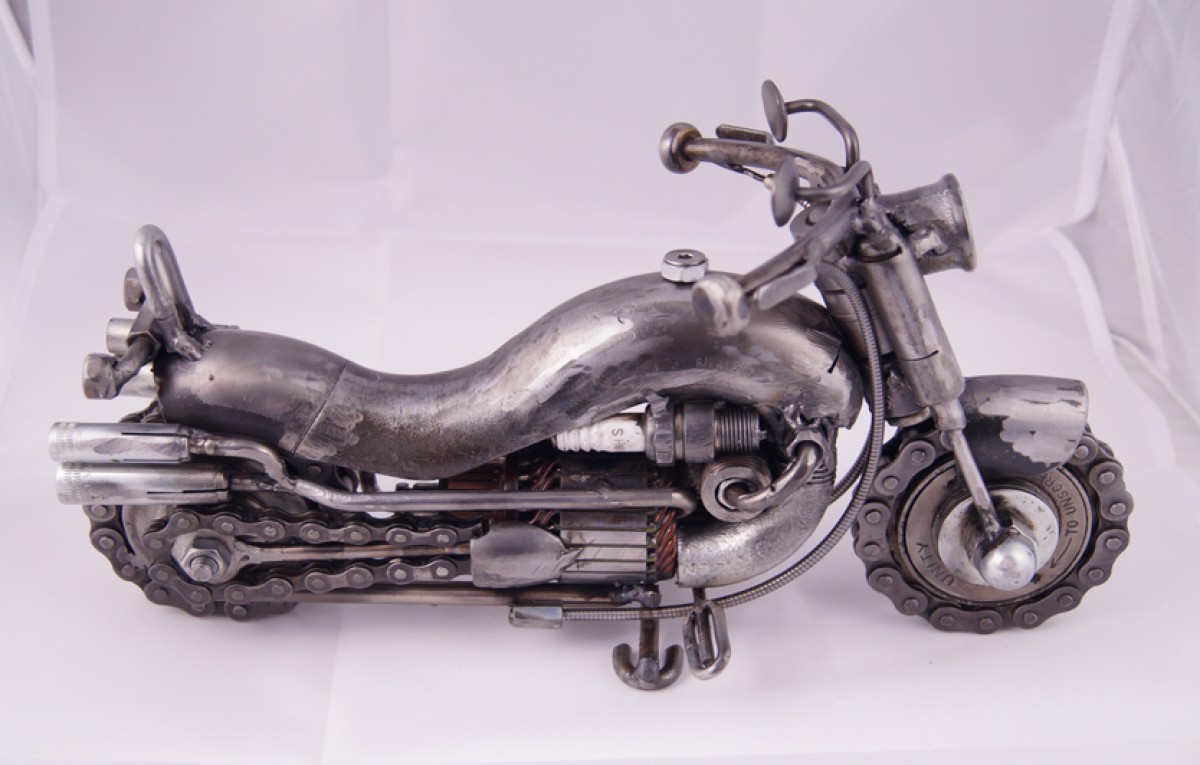The black and white photograph features a highly detailed, metal miniature model of a motorcycle against a white, wispy cloth backdrop. The motorcycle's frame is crafted entirely from various types of metal, giving it an industrial, gray steel appearance. Both the front and rear tires are uniquely fashioned from bicycle chains, resembling tank treads. The intricate design includes a chain running from the back tire to the motor area, indicating the bike's drive mechanism. Noteworthy features include metal handlebars, a small mirror extending from the front handlebar area, and a gas cap atop the curved seat, which is also made of metal. The model also depicts pedals, a kickstand, and a spark plug located beneath the gas tank, enhancing the realism. The exposed sections around the motor show either copper elements or rust, adding to the authenticity and giving a specific focus on the mechanical details. The motorcycle is positioned facing the right side of the image and has little to no cushioning, with the footrests and other components being solid metal.